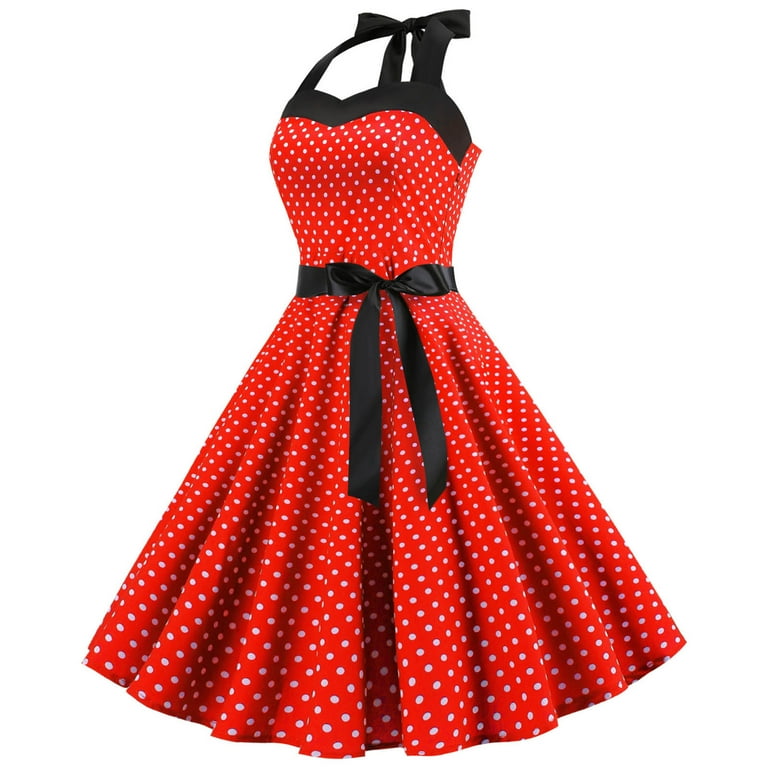The image showcases a vibrant, 1950s-style red dress adorned with small white polka dots. The dress features a fitted bodice with a flared, A-line skirt that creates a pleated look due to the abundance of material. A distinctive black sash, resembling a belt, cinches the waist and can be tied in a bow. The dress has notable black accents, including a black trim across the top of the bodice just above the bust, and black ribbon straps that tie behind the neck. The entire outfit is devoid of any background, set against a stark white backdrop, emphasizing the dress's vivid colors and classic design.